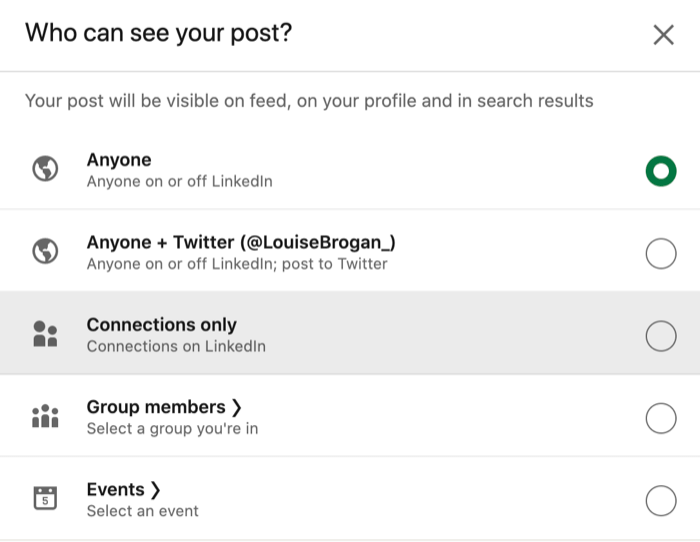**Detailed Caption:**

This screenshot appears to be a settings detail page on LinkedIn, titled "Who Can See Your Post?" At the top right corner, there is an 'X' to close the page. Below the title, there is a thin dividing line. The page explains, "Your post will be visible on feed, on your profile, and in search results." 

There are several visibility options provided:

1. **Anyone:** Indicated by a globe icon, this option means that anyone on or off LinkedIn can see the post. The radio button for this option is selected.
2. **Anyone + Twitter:** This option, also marked by a globe icon and noted with the text, "@LouiseBrogan_," suggests that the post will be visible to anyone on or off LinkedIn and will also be posted to Twitter. This radio button is not selected.
3. **Connections Only:** Represented by a people icon, this option restricts visibility to connections on LinkedIn. The radio button for this is not selected.
4. **Group Members:** Denoted by a group icon, this option allows visibility to members of selected groups the user is part of. It includes a right arrow to select the groups. The radio button here is unselected.
5. **Events:** Indicated by a calendar icon, this option allows the post to be shared with selected events, accessible via a right-arrow to select the event. This radio button is also not selected.

The chosen visibility setting is "Anyone" with the corresponding radio button clicked.